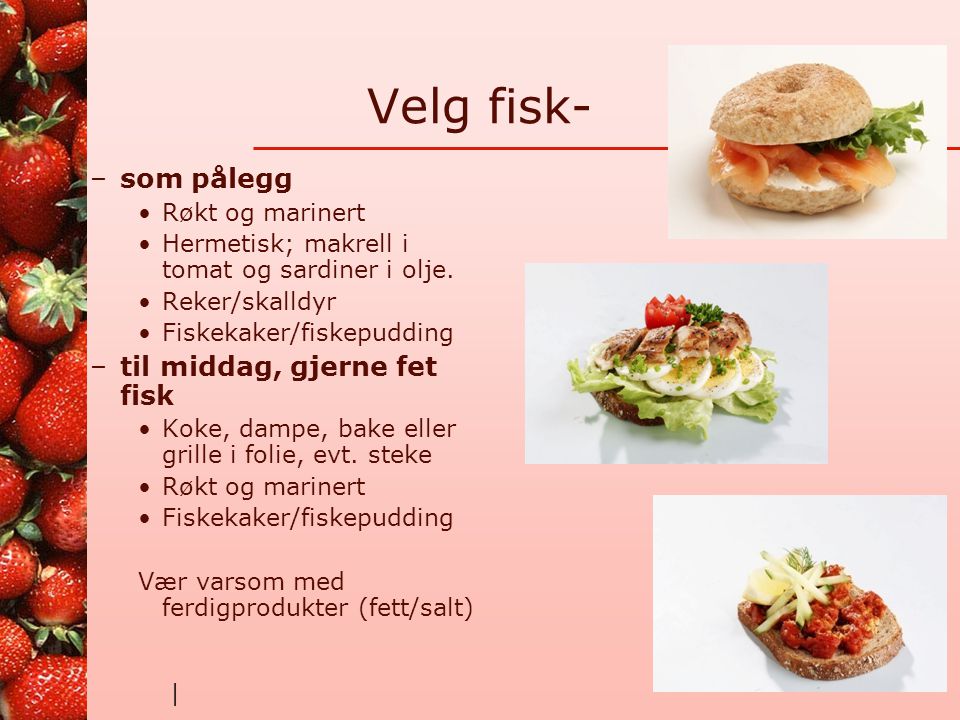The image features a food menu written in a foreign language, possibly German or French. The menu, adorned with a pink background, prominently displays the title "Velg Fisk" at the top center in dark brown text. On the left side, there is a vivid vertical strip showcasing fresh red strawberries with stems. The right side of the menu contains three food images. The top picture is a bagel with lettuce, fish, and cream cheese. The middle image depicts another bagel, this time topped with hard-boiled eggs, tomato, lettuce, and chicken. The bottom picture shows an open-faced sandwich with some kind of topping that might be cheese.